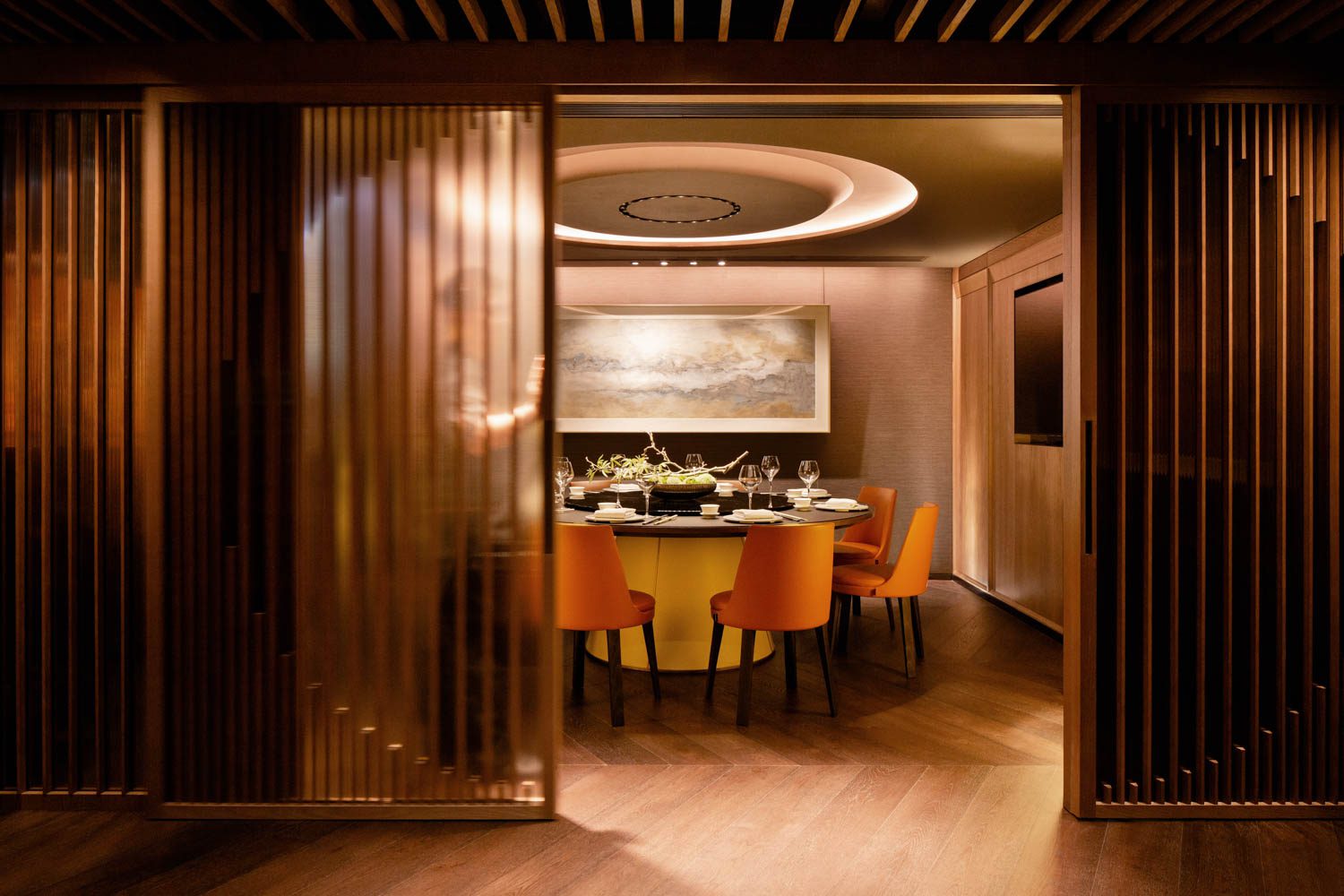The image depicts a private room in an Asian-inspired restaurant. Central to the room is a large, round table with a brown tabletop and a solid yellow base, furnished with a turntable for serving. The table is surrounded by orange chairs with black legs, set with white plates, napkins, and wine glasses, and features a centerpiece comprising tree branches, green elements, and a decorative bowl. The backdrop includes a lengthy, prominent painting of beach waves on the back wall, adding to the serene ambiance. Above, the ceiling hosts a round chandelier that illuminates the space warmly. The room's wood flooring extends to a sliding door with wooden slats, creating a partial transparency that allows a glimpse into the adjoining area where a man can be seen standing. This intimate dining area can be enclosed for a private dining experience.